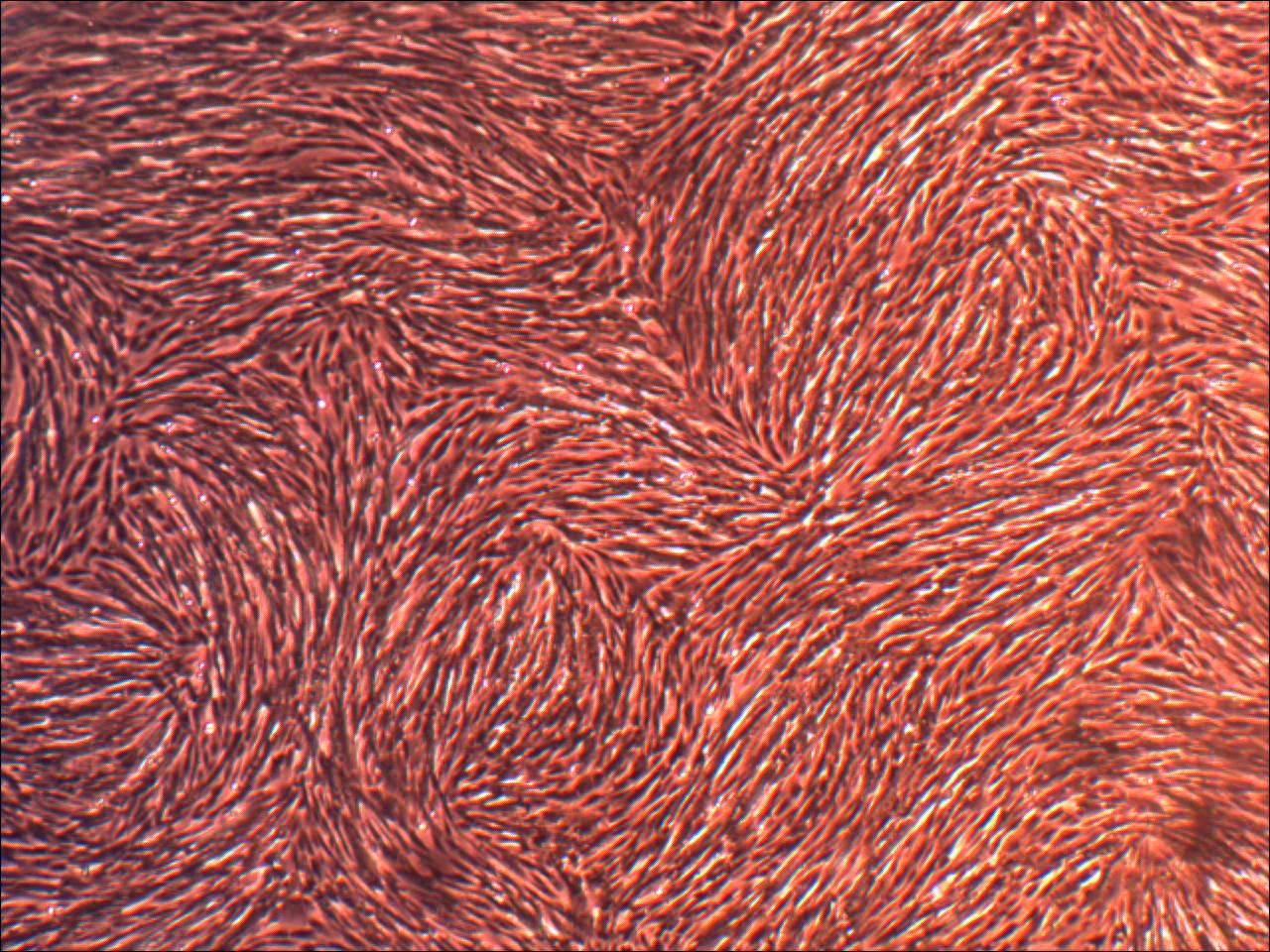This close-up image reveals a detailed texture of what appears to be a stringy or fibrous material. The primary color is a brownish-red hue, with lighter and darker areas that show where light hits and creates shadows in the crevices of the texture. Additionally, intermittent white fibers add diversity to the color pattern. The material, which is soft in appearance, resembles either yarn, fur, or a rug, characterized by short fibers that curve and swirl in various directions. The intricate pattern of these strands, flowing in multiple orientations—left, right, and horizontally—further enhances the complexity of the image. The lack of identifiable markers, such as text or signatures, emphasizes the abstract nature of this close-up fabric texture.